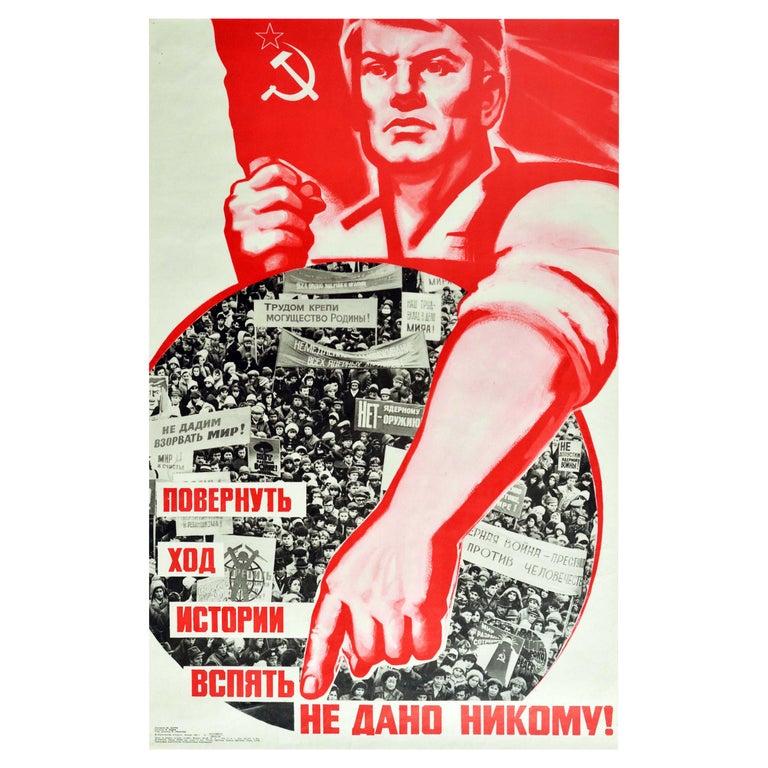The image appears to be a hand-drawn propaganda piece from the USSR. Dominated by a red background, it features a stern-looking man depicted in red with white skin and shirt, prominently holding the USSR flag in one hand. He gestures forcefully with his other arm extending over a large circle filled with a crowd of black-and-white figures, creating a stark contrast. These people, possibly representing a global populace, are depicted in a black-and-white photograph within the circle and hold banners with Russian text, possibly indicating protest messages. Above this assembly, there's a pronounced red headline in Russian on a white background, along with five text boxes also featuring Russian phrases, emphasizing the Soviet propaganda nature of the image. A hammer and sickle emblem is visible in the upper left corner, reinforcing its Soviet origin and intent.